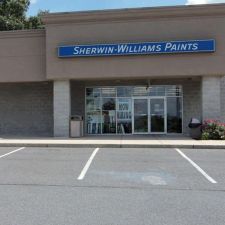Exterior view of a Sherwin-Williams Paints store on a clear day. The foreground features a building with a concrete brick base and an upper section clad in stone. The facade is accented by two prominent pillars that frame the entrance. Above the pillars, a blue sign with white lettering prominently displays the store's name: "Sherwin-Williams Paints." The front parking lot has two open spaces fully visible, with partial views of additional open spaces adjacent to them. The upper right-hand corner of the image reveals a backdrop of trees, a sliver of blue sky, and a few white clouds. Flowers are planted at the base of the right pillar, adding a touch of color to the scene, which also includes a trash can beside each pillar. The entrance consists of two doors, through which the store's interior lights and some items inside are faintly visible. Additionally, a "Now Hiring" sign is displayed in the window next to the doorway, inviting applicants.